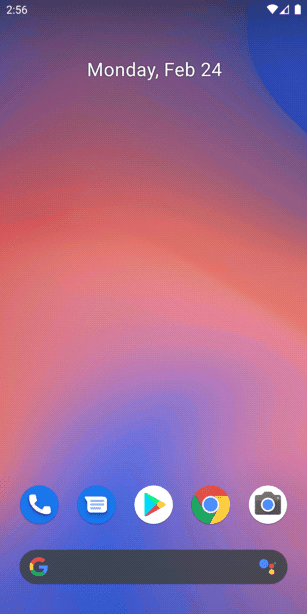The cell phone screen displays various elements in a neatly organized layout. In the upper left corner, the numeric indicator reads "256," while the upper right corner features icons indicating full Wi-Fi, cellular signal, and battery levels. Centrally positioned below these indicators, the date is clearly shown as "Monday, February 24th."

At the bottom of the screen, a row of five icons sits aligned from left to right: the Phone app, Text messages, Play Store, Google, and Camera. Beneath these icons is a prominent Google search bar set against a black background, showcasing the Google 'G' logo in its distinctive red, yellow, green, and blue colors. To the right of the search bar are smaller blue, red, green, and yellow circles, likely representing Google's AI logo.

The wallpaper of the screen is an eye-catching gradient that transitions from blue at the bottom to a purplish hue, then pink, followed by yellow, light orange, orange, and back to pink, purple, and blue towards the right corner. 

The various icons on the screen exhibit a color palette comprising blue, green, yellow, red, white, black, and gray, predominantly reflecting Google's signature colors interspersed with basic shades of black, white, and gray.